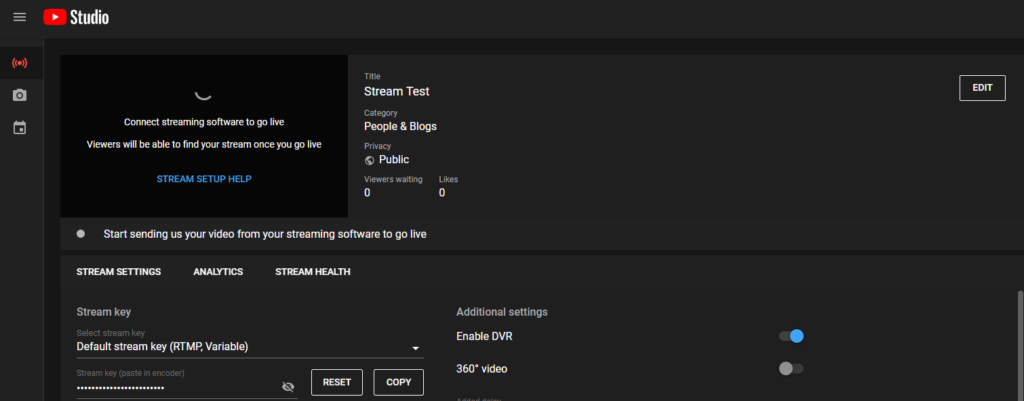Screenshot of a Livestream Setup Interface

The image is a screenshot of a computer screen showcasing a livestream setup interface. The layout is predominantly black with contrasting white text. 

In the upper left corner, the word "Studio" is displayed in white. Adjacent to it, there's a red rectangle featuring a white arrow, indicative of a clickable button. 

A black rectangle below contains a message: "Connect Streaming Software to go live. Viewers will be able to find your stream once you go live." A blue hyperlink reading "Stream Setup Help" is also present within this rectangle.

To the right of this section, several details about the stream are outlined:
- Title: Stream Test
- Category: People and Blogs
- Privacy: Public

Directly below the black rectangle, there's another informative message next to a white circle icon. The message reads: "Start sending us your video from your streaming software to go live."

Further down the interface, the following tabs are mentioned: Stream Settings, Analytics, and Stream Health, suggesting monitoring and configuration options.

In the upper right corner of the screenshot, there is an "Edit" button inside a small rectangle, allowing for further adjustments to the stream setup. The overall context indicates that the website or application is designed for managing and broadcasting livestreams.